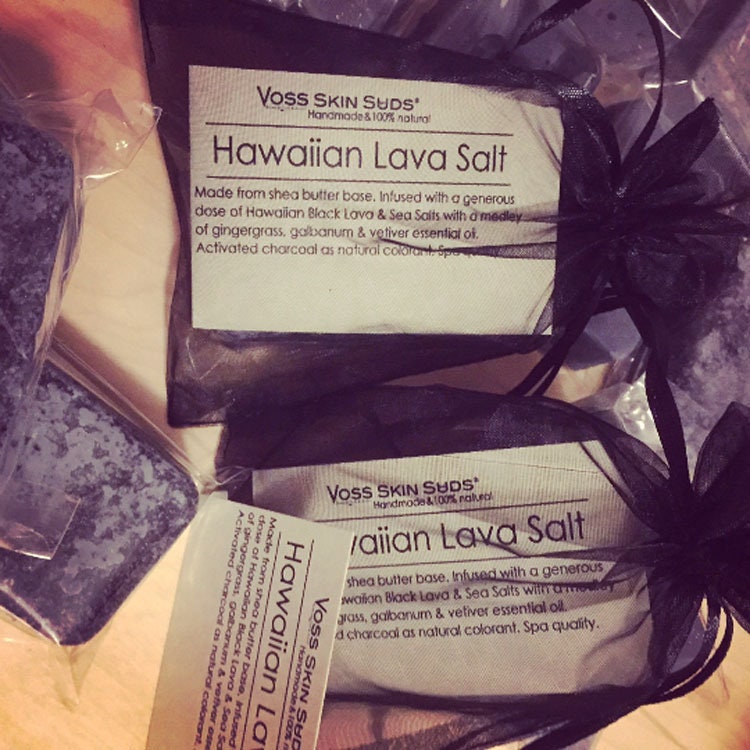In this image, there are two charming gift bags positioned parallel to each other, made of a purple mesh material. These bags are tied at the top with a little ribbon and twine, creating a cute poof effect. Inside each bag, visible through the mesh, is a large cream-colored label that reads "Voskin Suds, handmade, 100% natural." The label further describes the contents: "Hawaiian Lava Salt, made from a shea butter base infused with a generous dose of Hawaiian black lava and sea salts, with a medley of ginger grass, galbanum, and vetiver essential oils, and activated charcoal as a natural colorant, spa quality." To the left of these mesh bags are a couple of bars of soap wrapped in plastic. The soaps have a purple hue with some grayish tones. Additionally, there appears to be an assortment of similar little goodie bags displayed in the upper right-hand corner of the image.